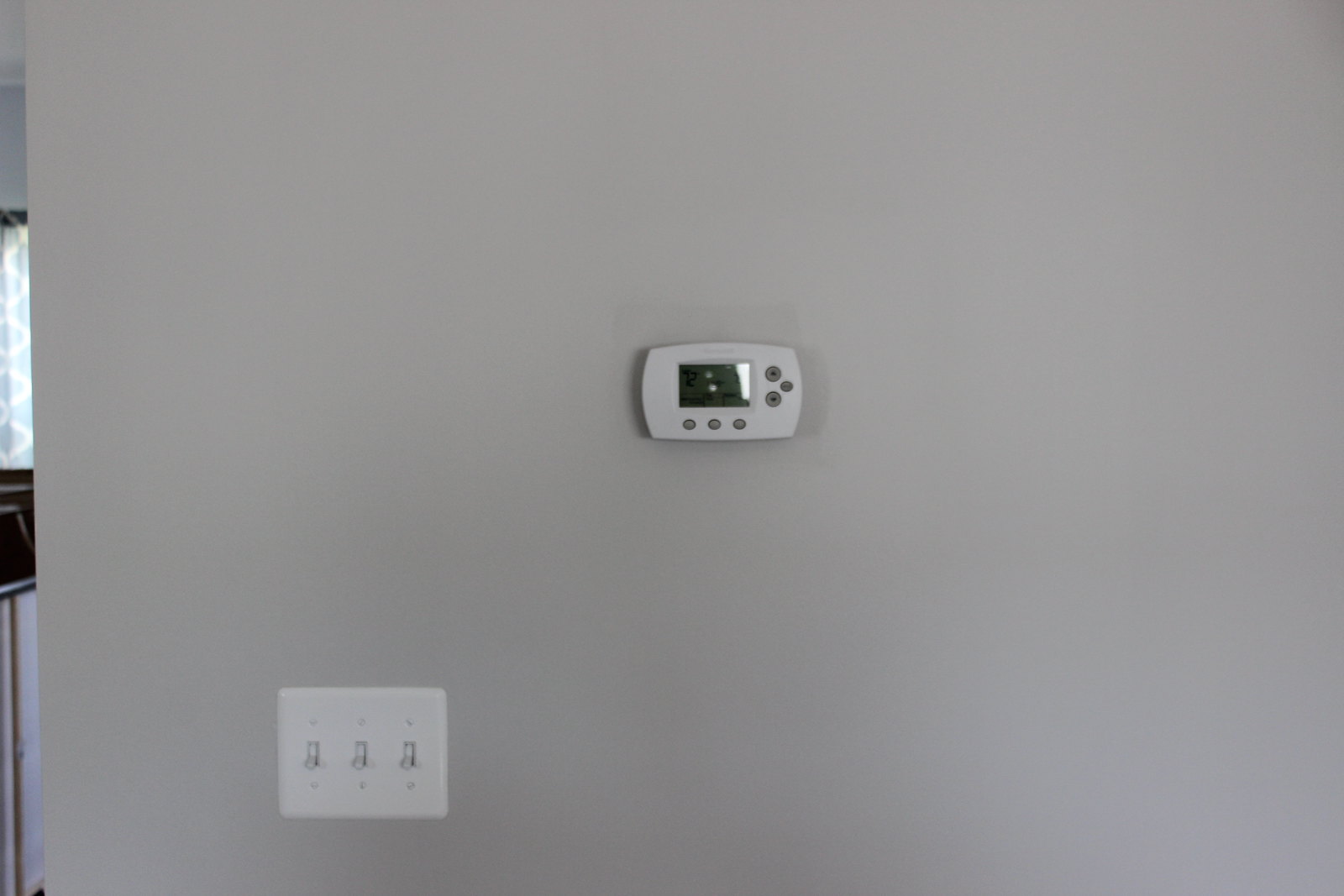This landscape-oriented photo captures an interior wall of a home, painted in a neutral light gray or tan hue typical of fiberboard materials. Illuminated by what appears to be natural daylight, the image showcases two prominent fixtures mounted on the wall. Centrally positioned is a programmable thermostat, displaying a temperature setting of 72 degrees, with a casing that matches the off-white color of standard home fixtures. In the lower left section of the photo, a trio of light switches is grouped together on a single off-white outlet cover. All three switches are in the down position, suggesting they are currently turned off. The overall composition and lighting of the photo contribute to a calm, orderly aesthetic.